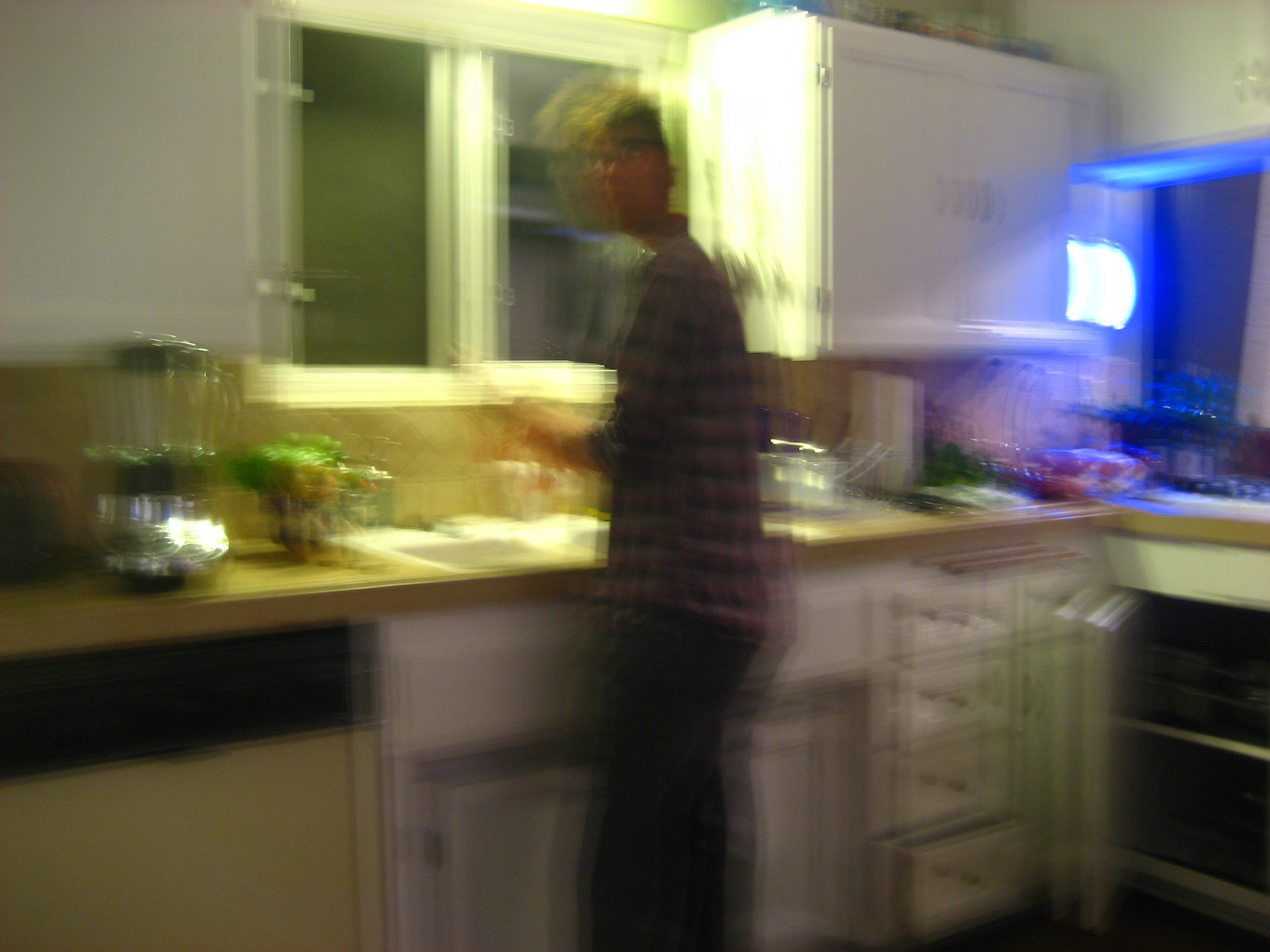In the center of the image, there's a kitchen square workspace. At the far end, a dark window provides a backdrop, covered in a black shade. To the right, a sleek white cabinet with polished handles stands out, extending upwards. On the left side of the image, a pristine white wall is visible. The countertop is adorned with a textured backsplash made of tiles. A blender and mixer are positioned on the left-hand side of the counter. Below the countertop, wooden cabinets and drawers provide storage. On the right-hand side, a series of vertical drawers line the space. A slightly out-of-focus person is standing within the scene. In the upper right corner of the image, a blue light casts a cool, soft glow, illuminating part of the area.